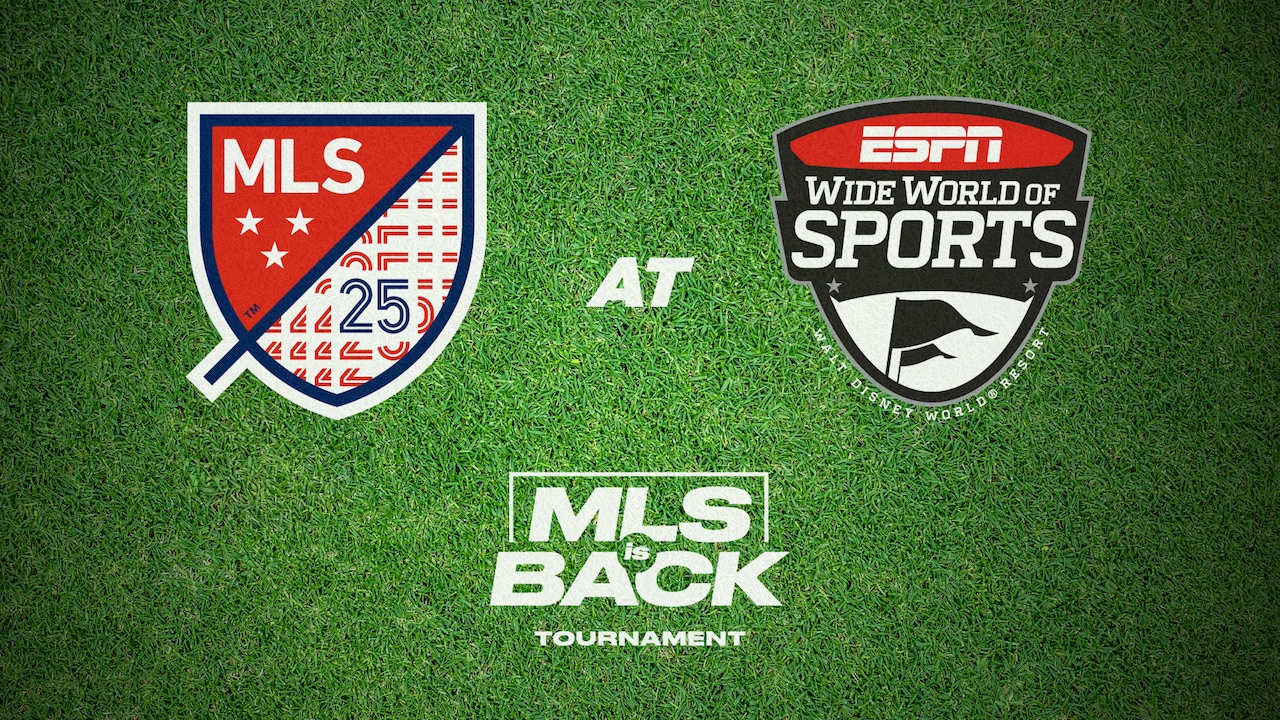The image is a close-up of a green grassy area, likely astroturf, resembling a sporting field. The background features a radial gradient, bright green in the center fading to darker green towards the edges. In the center of the graphic, there are two prominent emblems positioned side by side.

On the left, there's a shield-shaped logo divided diagonally from the top right to the bottom left. The top half of this shield is solid red with white capital letters "MLS" and three white stars underneath. The bottom right section of the shield features a blue number "25" with red echoes.

On the right, there's another emblem with a bowed top. The topmost section of this emblem displays the ESPN logo in white against a red background. Below it, in the black center, "Wide World of Sports" is written in white letters, and the bottom section is white with two black flags and the text "Walt Disney World Resort."

Between the two emblems is the word "AT" in white. At the bottom center of the image, in large white lettering, it reads "MLS is Back Tournament." The overall design suggests an advertisement for a sports event, combining elements from Major League Soccer and ESPN's Wide World of Sports.